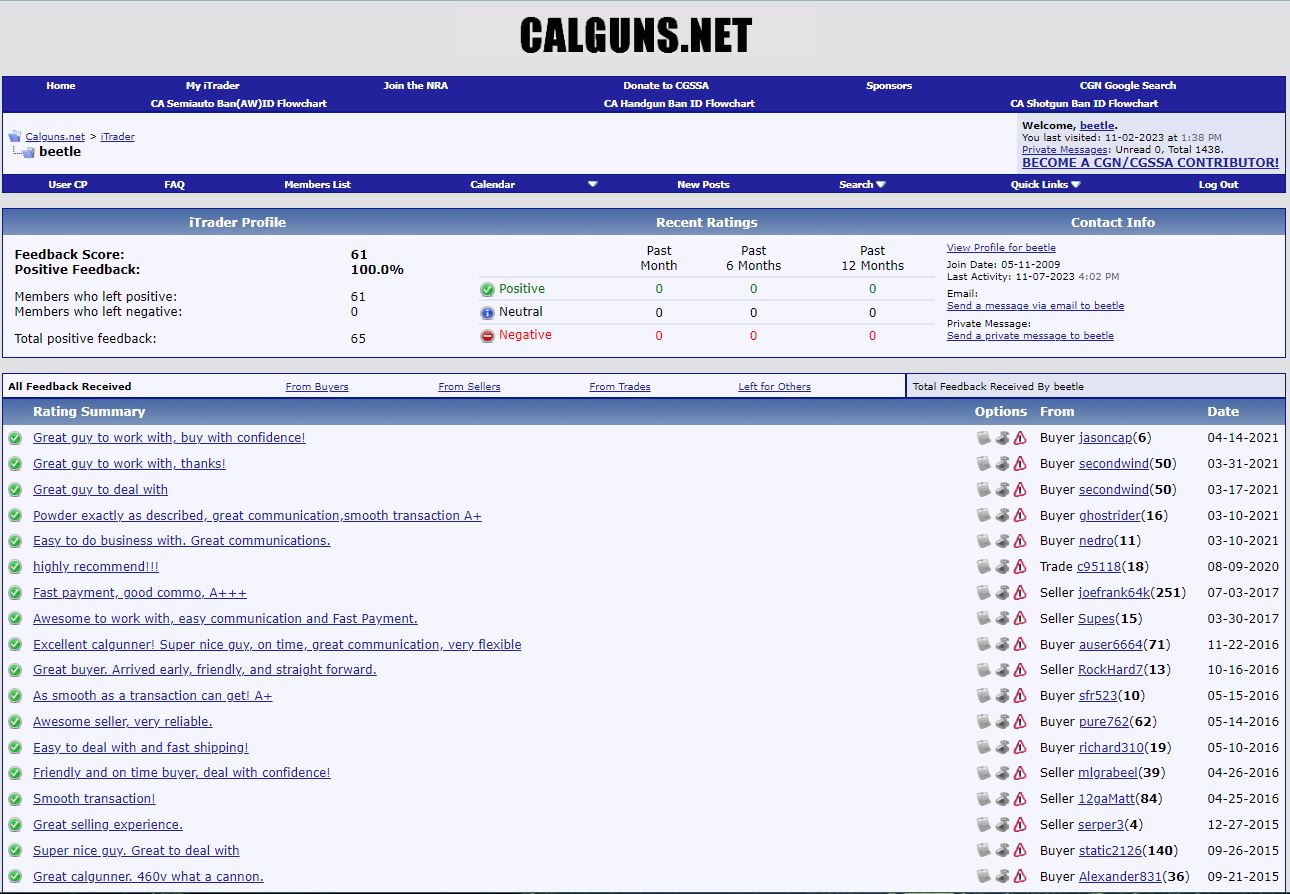The image depicts the interface of the Calguns.net forum, specifically showcasing the user feedback section. At the top, there is a wide horizontal gray bar with the site's logo, "Calguns.net," prominently displayed in the center. Below this bar, there is a blue and white box containing various navigational tabs such as Home, My iTrader, Join the NRA, Donate, Sponsors, CGN Google Search, User CP, Frequently Asked Questions, Member List, Calendar, New Posts, Search, Quick Links, and Log Out. 

Further down, we find the user’s iTrader profile showcasing a 100% positive feedback score. The profile includes sections for viewing recent ratings and detailed feedback. The feedback interface is divided into various tabs: From Buyers, From Sellers, From Trades, and Left for Others. Below these tabs is a rating summary, showing detailed options for the user, date sections, and a long list of feedback entries. All feedback entries feature a green check mark to the left, indicating positive feedback.